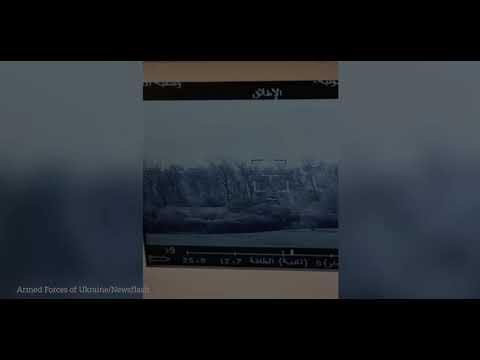This small, dark, and grainy photograph presents a challenging view that appears to depict an outdoor setting dominated by a mountain range or rock formation against a blue sky. Below this formation is a dark bluish-green area, potentially either a meticulously maintained grassy expanse or a river. The scene is framed in the foreground by a wide, dark brown half-brick wall with white mortar, and a paved road lies just beyond it. The photograph is almost square, with a highlighted center displaying blurred imagery—possibly a war-torn city—hinted at by pixelation and grayscale tones. Across this image, white Arabic text overlays a black bar at the top, while a similar black bar at the bottom includes a rocket symbol and distance markers. English text in the bottom left corner clearly states, "armed forces of Ukraine," lending a sense of context and perhaps gravitas to the captured moment.